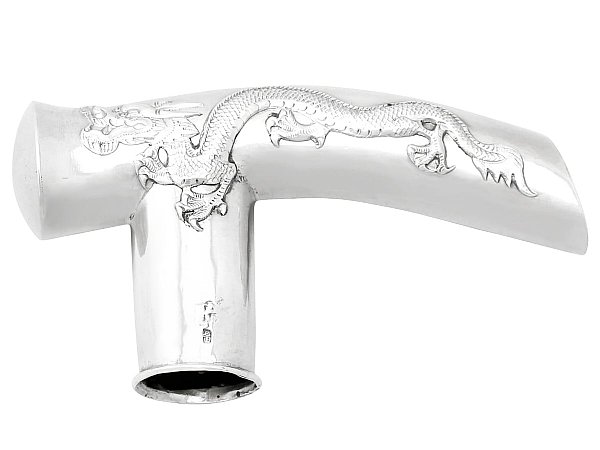The image is a horizontal, borderless photo depicting what is likely the handle of a cane. The elaborate silver handle features a detailed etching of a mythical dragon resembling the Asian-style depiction, with two heads and four feet. The dragon's intricate scales and fierce expression, complete with teeth and extended claws, wrap around the handle from left to right. The lower stem of the handle, which is open at the bottom, includes small indents that appear to be Asian letters. The background is plain white, emphasizing the striking contrast and detail of the shiny, ornate design.